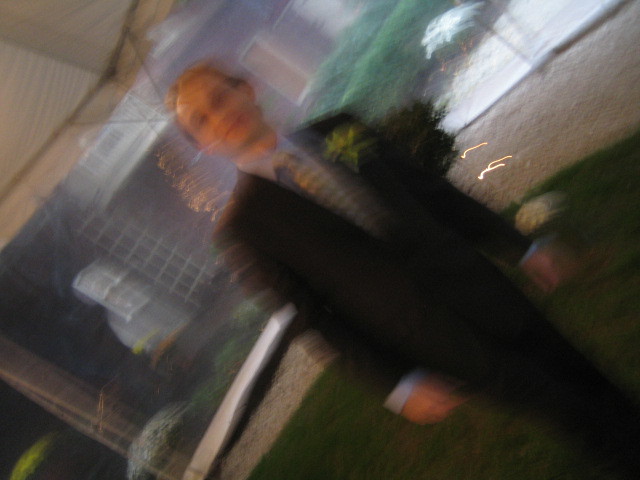The photograph, though very blurry and out of focus, captures an outdoor scene featuring a man standing on a grassy area under a large white tent. He is wearing a dark, possibly black or dark gray suit complemented by a light blue dress shirt and a tan or yellow tie. A small yellow flower boutonniere adorns his lapel. The man, who has a fair complexion, a bald spot, and a slight smile, is seen tilting slightly to the left due to the photo’s angle. Behind him, there are hedges and a house with a distinct purple color and a white balcony at the top. Despite the motion-induced blurriness, the setting appears to be calm with planted areas and shrubbery visible through the glass windows or openings. The scene seems to capture a moment of waiting or pause, giving a glimpse into a festive or formal occasion in an outdoor but partially enclosed space.